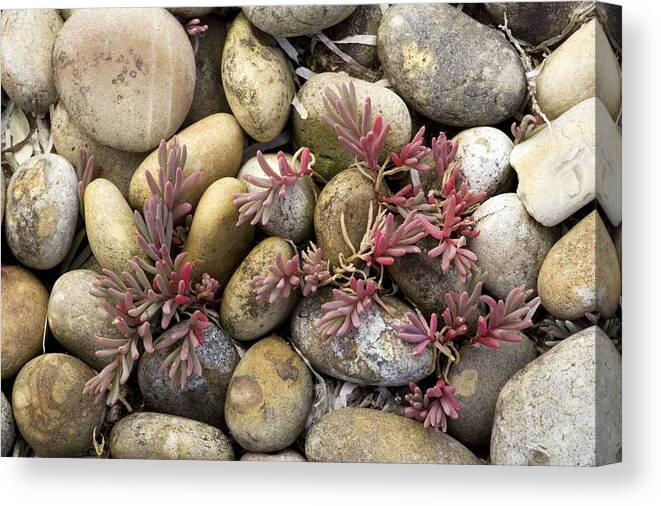The image depicts a ground fully covered with a diverse array of smooth, round to oblong rocks in various colors—ranging from beige and yellowish-beige to light gray, almost white, and some darker shades. The rocks vary in size, with some weighing approximately 5 pounds and others as light as 2 pounds. Among the rocks, various plants are sprouting, which resemble succulent leaves. These plants have long, slender leaves with a mix of pinkish-purple, brownish, red, and green hues. Toward the top right of the image, there are some square-shaped rocks and spaces with visible dirt, where it looks like ribbons might be intermingled. On the far left top, there’s a larger off-white rock, appearing to have some dirt that almost looks like writing. The arrangement of rocks and plants gives the scene a carefully curated, artistic impression, highlighting the interplay of natural textures and colors.